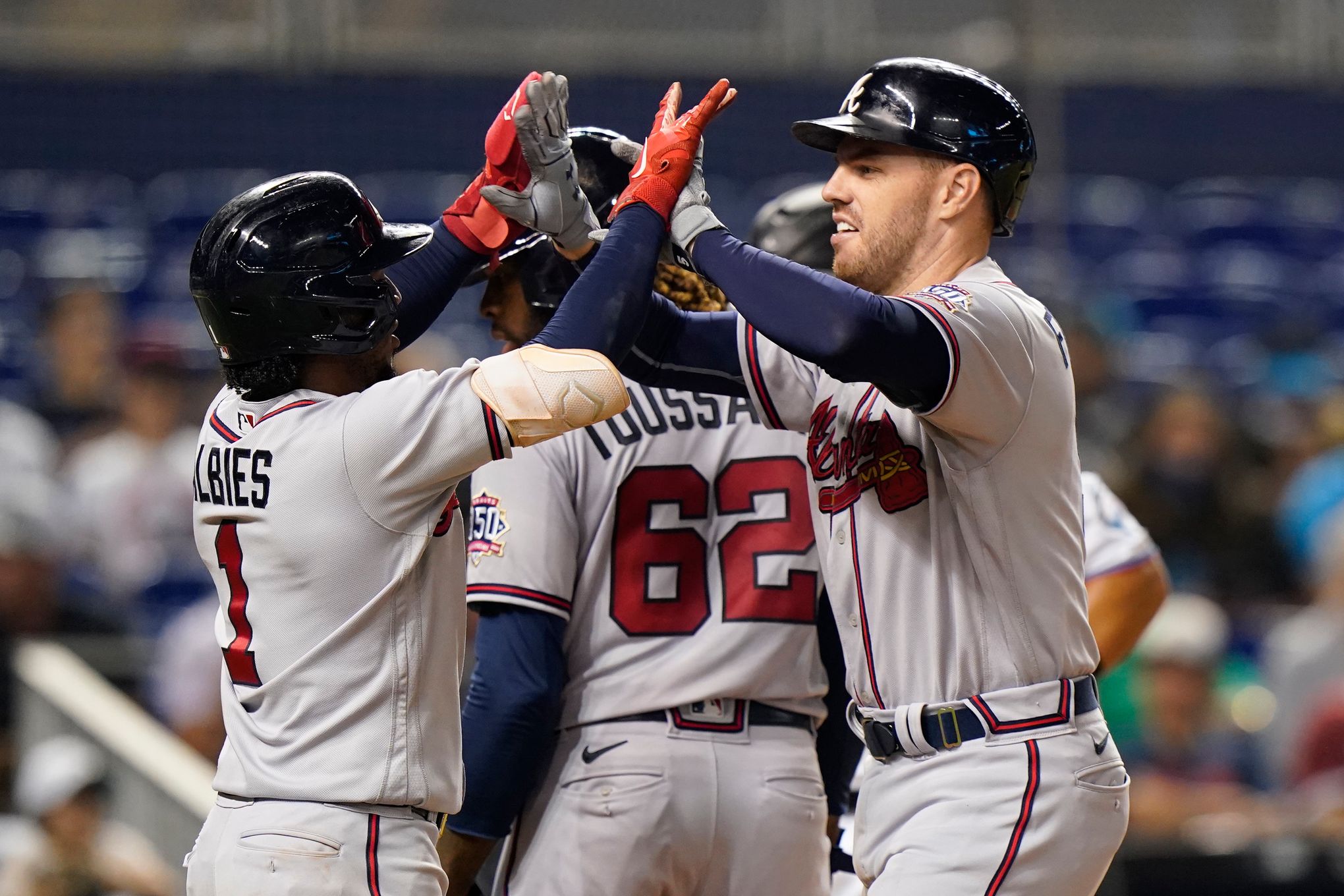In this realistic, horizontally oriented photograph, a jubilant scene unfolds at an Atlanta Braves baseball game. The image prominently features two players in the foreground, both with smiles on their faces, wearing the Braves' gray away uniforms with the distinctive burgundy "Braves" logo and an axe below the name. The player on the left, identified by "Albies" and the number 1 on his jersey, is shown wearing a guard on his elbow and red gloves, while high-fiving a white teammate on the right, both of whom are sporting black belts and helmets. The background, slightly out of focus, reveals stadium seats in blue with a small crowd dispersed among them and the barely discernible elbow of an umpire. There are additional Braves players in the middle ground, all seemingly sharing in the high-spirited moment. The stadium appears partially filled, enhancing the intimate yet victorious atmosphere.